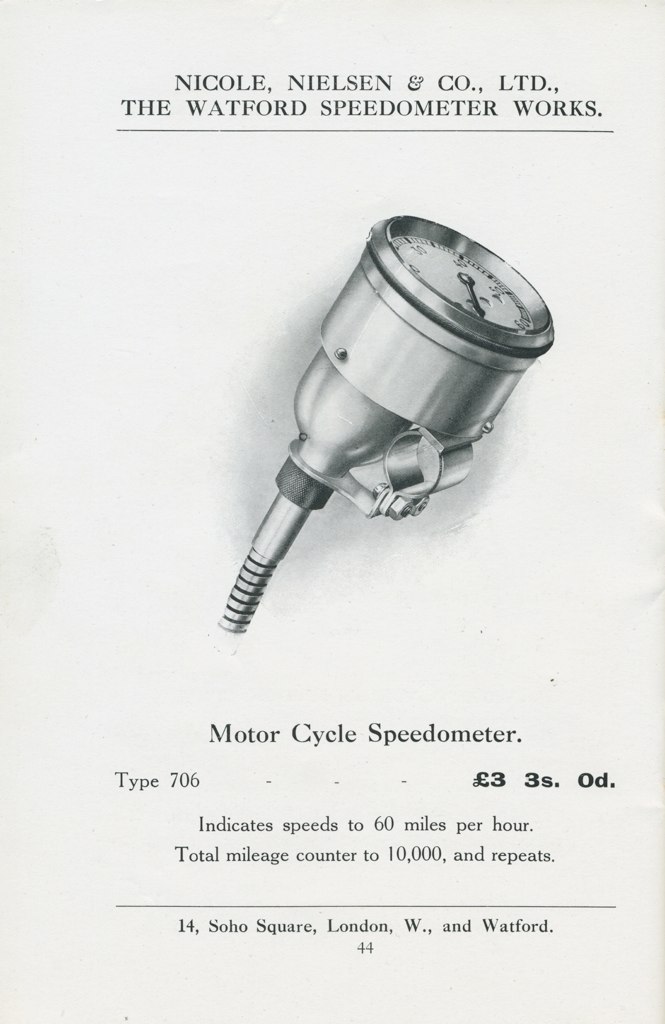The advertisement features a detailed illustration of a motorcycle speedometer. At the center of the white paper lies a meticulously drawn silver gauge with a circular base, connected by a slender silver cord. The face of the gauge is enhanced with numerals and a precise black needle. Above the image, the text reads "Nicole Nielsen, ENCODE, LTD – No wait for it, speedometer works." Below the gauge, additional details specify "Motorcycle Speedometer, Type 706," capable of indicating speeds up to 260 miles per hour and counting total mileage up to 10,000 miles before repeating. Soft gray shadings subtly highlight the center, giving a delicate contrast that enhances the visual appeal of the shiny, compact speedometer illustration.